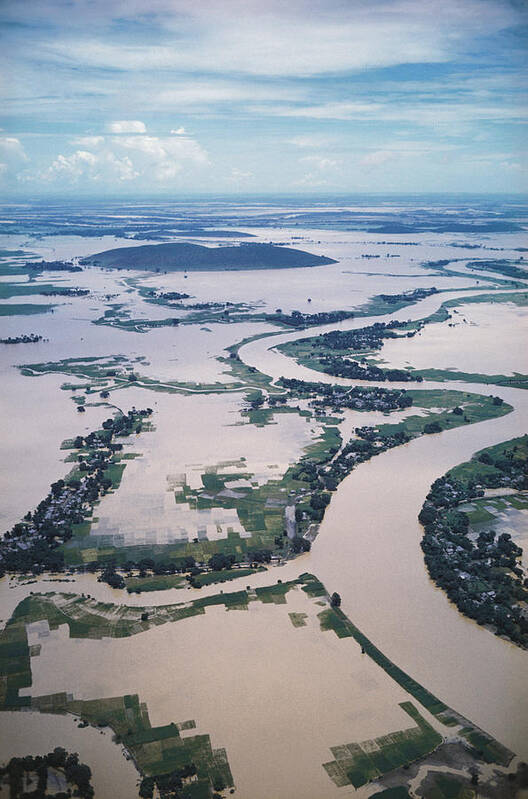This is a photograph, taken in portrait orientation, which provides a bird's-eye view of a river experiencing significant flooding. The river, which is a murky brown, has overflowed its banks and inundated the surrounding areas, including fields, farmlands, and patches of green grass. These green patches break up the expanse of beige, flood-affected land, highlighting the extent of the water's reach. Nestled in the backdrop, a mountain or large hill is partially surrounded by water. The landscape is devoid of buildings, suggesting they might have been submerged or are not visible in this particular region. Above this flooded terrain, the sky contrasts with a bright shade of turquoise, dotted with clusters of white clouds. The overall scene captures a dramatic and expansive view of land coping with severe flooding.